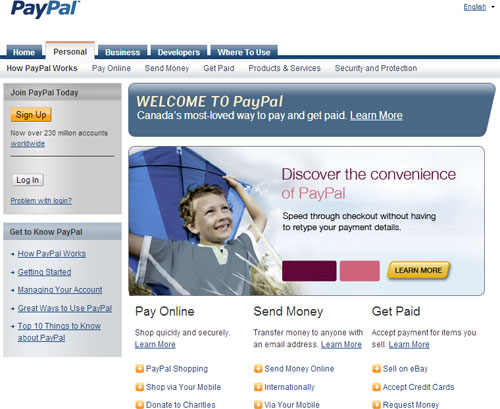The image showcases the PayPal website, prominently featuring the PayPal logo in the top left corner. Towards the top right, there is an option to change the site language, which is currently set to English. Beneath this, a navigation menu includes several tabs: Home, Personal, Business, Developers, and Where to Use, with the Personal tab currently selected. 

Under the Personal tab, various sub-sections are listed: How PayPal Works, Pay Online, Send Money, Get Paid, Products and Services, and Security and Protection. The "How PayPal Works" section is highlighted in black and slightly bolded, indicating it is the current selection.

The left side of the screen features headings such as "How You Can Join PayPal Today," accompanied by an orange Sign-Up button and a grey Log-In button for existing users. Below these buttons, there is general information guiding users on how to familiarize themselves with PayPal.

On the right side, a blue banner welcomes users to PayPal, showing a smiling young boy next to purple text that reads, "Discover the Convenience of PayPal." Below this text is a yellow "Learn More" button for additional information. Further down, the page is divided into three sections with headings: "Pay Online," "Send Money," and "Get Paid," each with various clickable sub-headings for detailed exploration.